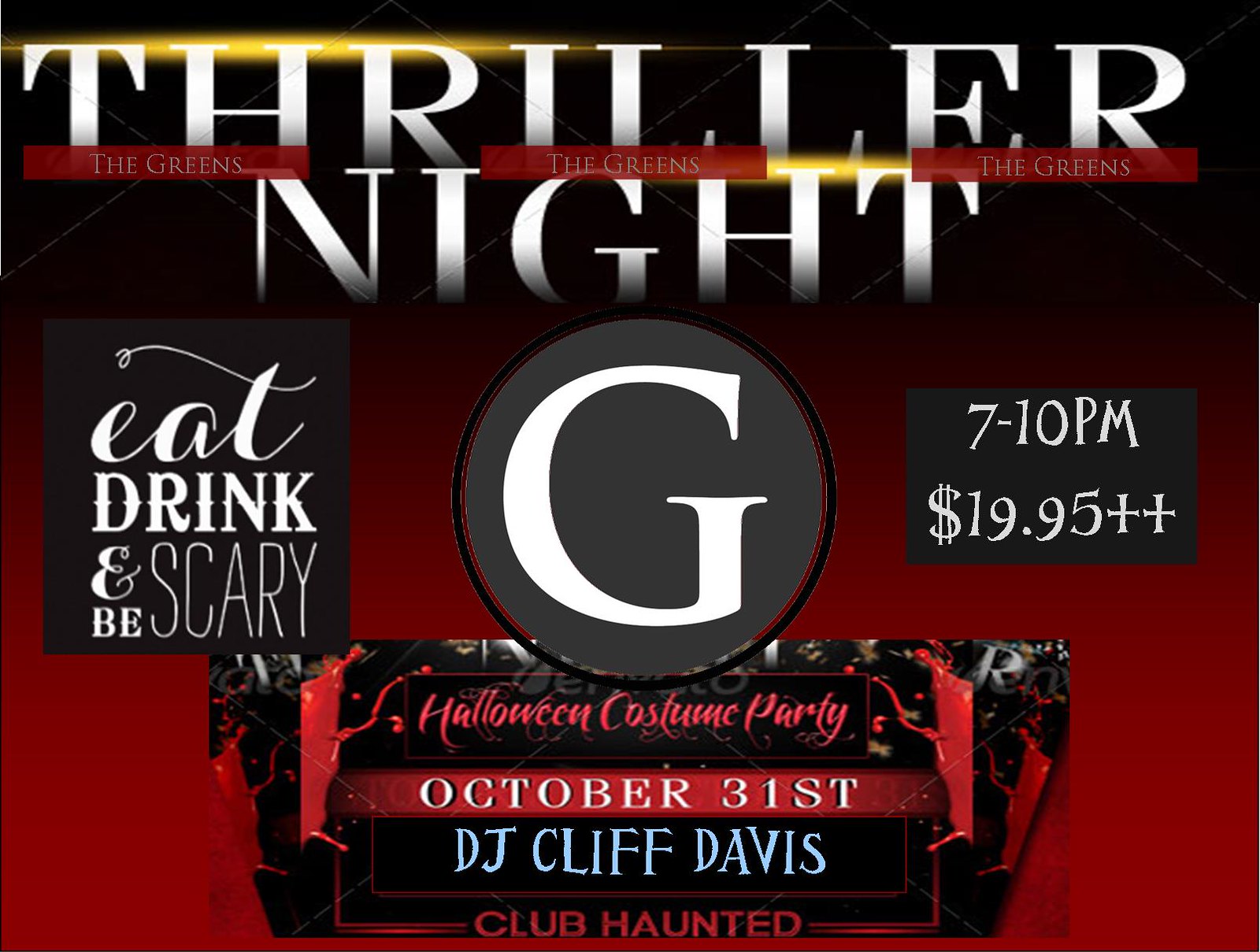The image appears to be a promotional flyer or poster for a Halloween event with prominent graphic design elements. Set against a predominantly black background with red accents, the focal point at the top features the bold white text "Thriller Night," highlighted by diamond shapes and red rectangular blocks interspersed between the words.

Prominently displayed throughout the image is the repeated phrase "The Greens" in a silver-gray font—one instance each on the left, middle, and right sides of the upper section. The central element of the design is a gray circle housing a large white "G," bordered by a blend of black and red. To the left of this circle, a white text box within a red-splattered, black square reads, "Eat, Drink, and Be Scary." 

To the right, contained within a gray rectangle, the details "7 to 10 p.m." and "$19.95" followed by two white crosses are clearly visible. Below these elements, the flyer continues with additional graphic flourishes, including red blood splatters extending towards the edges. 

In the center, red text against a black background announces, "Halloween Costume Party," flanked by the date "October 31st" in white on a red background. Beneath this, white text on black advertises "DJ Cliff Davis," and at the very bottom, "Club Haunted" is prominently featured in red text against a black background, tying all elements together with a cohesive red backdrop. The overall design exudes a spooky, thrilling atmosphere befitting a Halloween celebration.